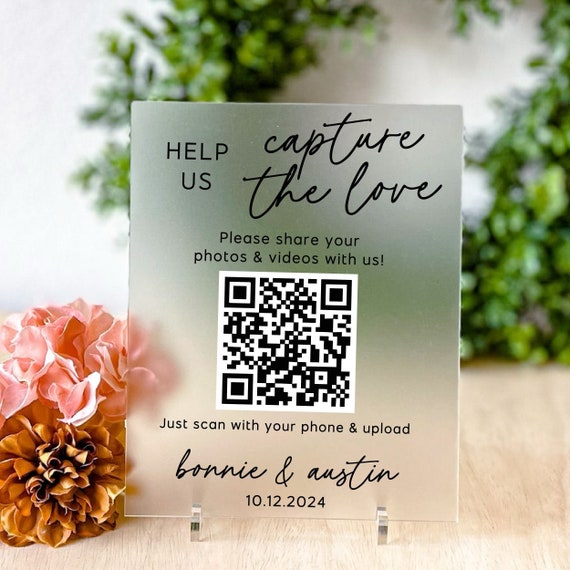The image depicts a clear, frosted acrylic sign mounted on a sleek silver stand situated on a light blonde woodgrain table. To the left of the sign, there are beautiful pink and tan roses, adding a romantic touch to the scene. In the background, against a white wall, a green leafy wreath can be seen, though out of focus.

The sign itself features a black QR code with the following text: "Help us capture the love. Please share your photos and videos with us. Just scan your phone and upload." The phrase "Help us" is in regular black print, while "capture the love" is elegantly scripted in cursive. Below the QR code, the text reads "Bonnie and Austin," with the date "10-12-2024" inscribed in a handwritten style.

This wedding prop invites guests to easily share their captured moments by scanning the QR code, allowing Bonnie and Austin to collect cherished memories from their special day.